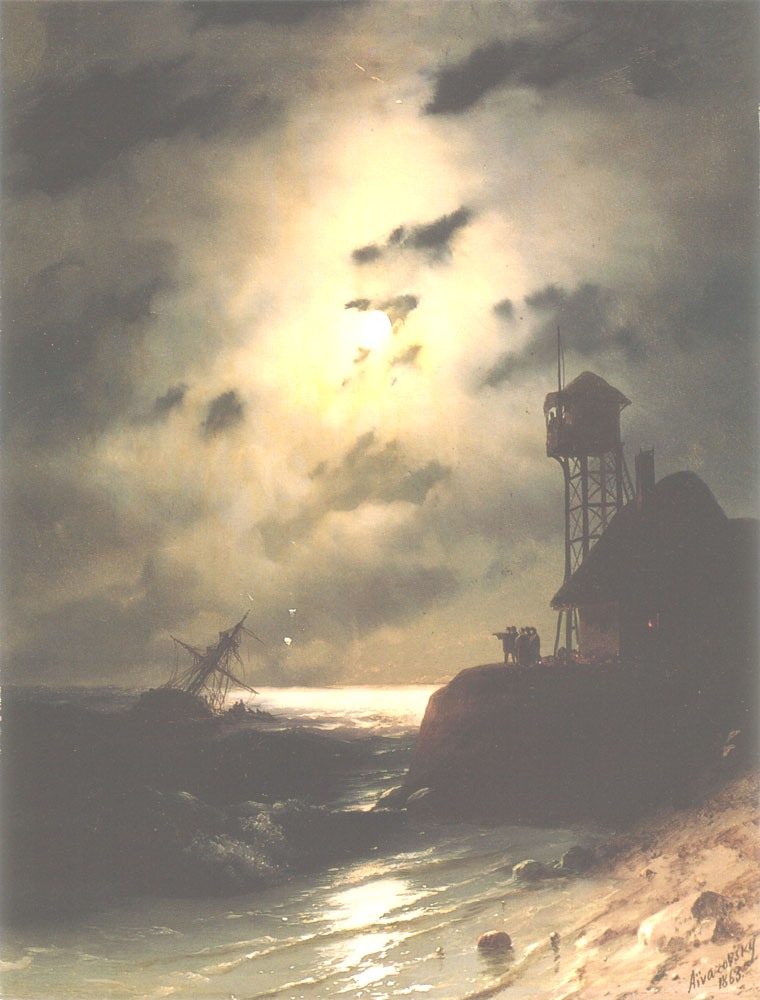This detailed oil painting, titled and signed by Eva Nowitzki in 1868, captures a dramatic nocturnal scene by the ocean. The darkened setting is illuminated by the moon peeking through storm clouds, casting a reflective glow onto the turbulent waters below. Central to the composition, a ship in distress lists heavily to starboard, appearing on the verge of capsizing. This vessel, evocative of an 1800s shipwreck, dominates the lower left-hand corner, its fate seemingly sealed by the relentless waves.

To the right of the moon, a small gabled structure resembling a wooden lighthouse stands tall on a cliff, accompanied by a sturdier building with walls, a gabled roof, and a chimney, probably serving as a keeper's house. A group of people can be seen in front of this house, pointing towards the doomed ship, adding a human element to the scene.

The foreground features a sandy beach with waves gently lapping the shore, forming a stark contrast to the peril faced by the ship. The meticulous detail captures not just the physical elements, but the palpable tension and drama of the stormy night. The artist's signature, 'Eva Nowitzki, 1868,' is distinctly visible in the bottom right-hand corner, affirming the painting's historical context and artistry.